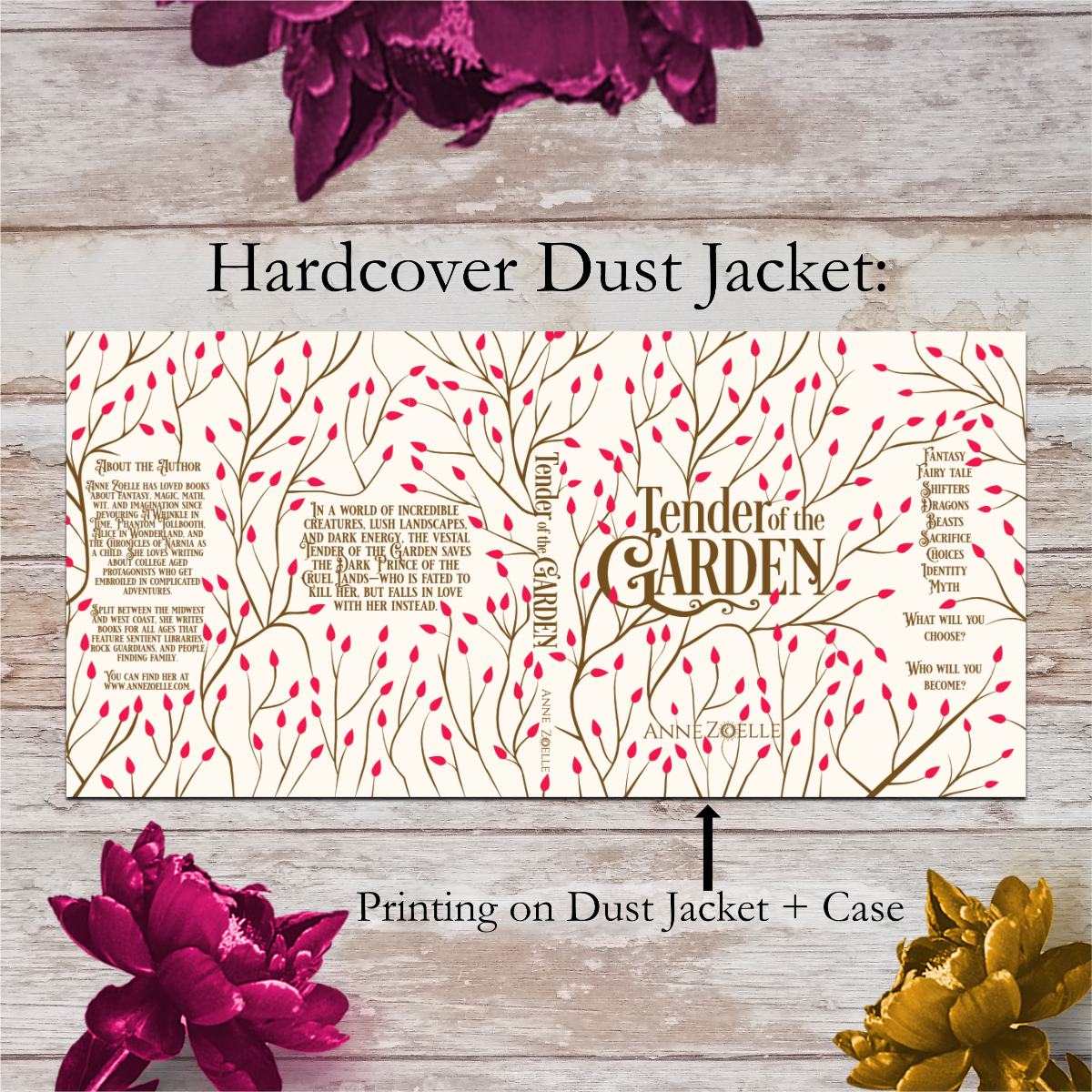This image presents a detailed layout of a hardcover book and its dust jacket. The setting is a wooden plank background, with the book positioned centrally. The wood features white and gray linear patterns, enhancing the contrast with the book. At the top of the image, a purple flower dangles above the book, while at the bottom left rests another purple flower and to the bottom right, a gold-hued flower. 

The hardcover book is predominantly beige with green-stemmed, pink flowers adorning its surface. "Tender of the Garden" and "Zoe" are inscribed vertically in the middle of the book's cover. The dust jacket cover features intricate vine designs with red, tulip-like flowers on its edge. "Tender of the Garden" appears again across the jacket spine in a light black-gray text, while on the right side of the book, the title and author's name are repeated in darker brown text, oriented horizontally.

To the left side of the image, there are paragraphs of text about the author, though the specific details remain unreadable in the current view. An arrow pointing upwards towards the hardcover directs attention to the note, "Printing on dust jacket + case," written in black font. This arrangement highlights not only the aesthetic elements of the book and its cover but also emphasizes the detailed engravings and design components from various perspectives within the image.